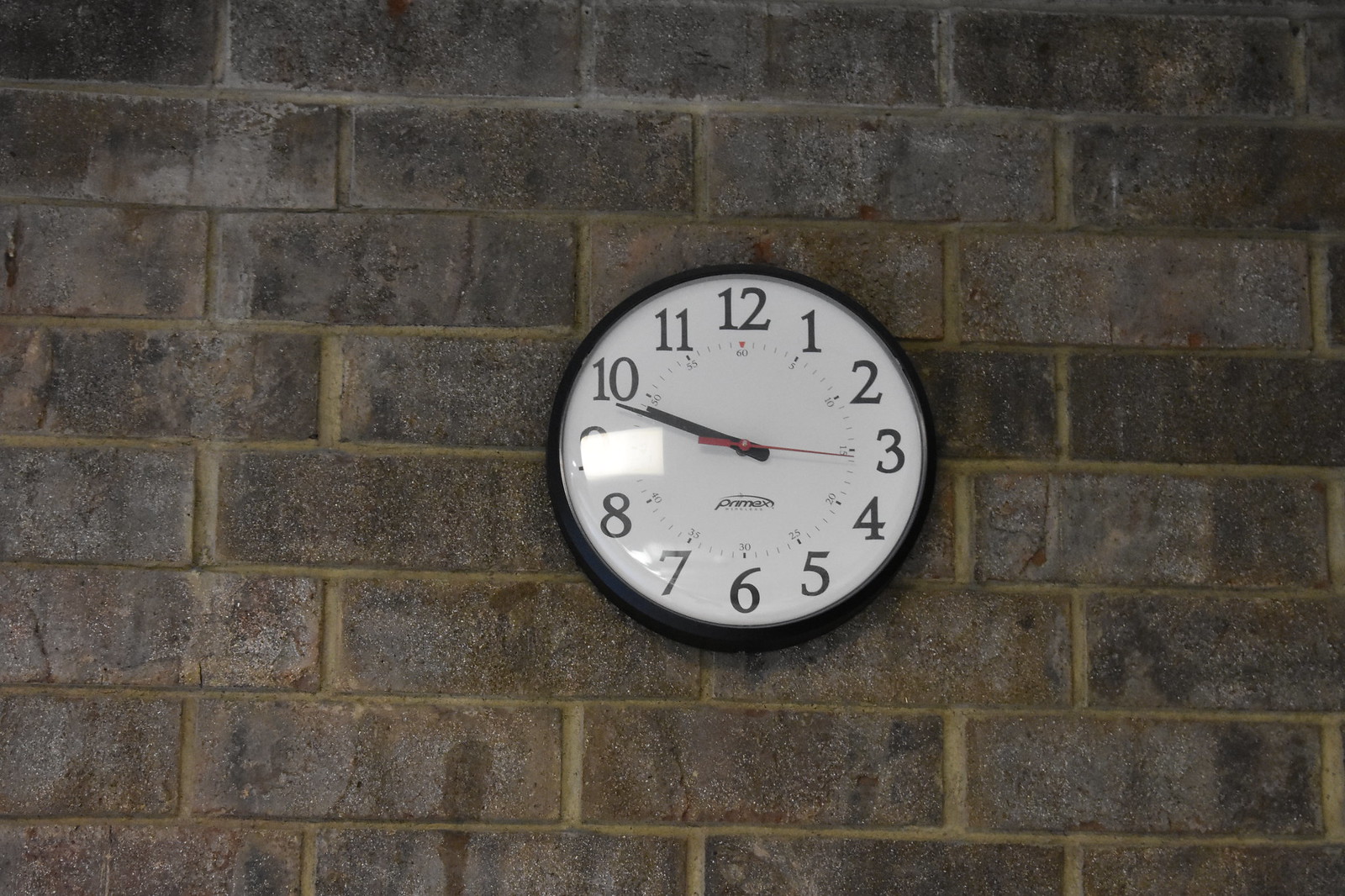A round clock with a black border is mounted on a rugged stone brick wall. The clock face displays the numbers 1 through 12 around its circumference, with two black hands indicating that the time is approximately 9:48. A red second hand points to just below the 3, marking roughly 15 seconds. The clock features the logo "Primex" on its surface, accompanied by a distinctive swoosh that arcs from the X over the top of the word. Additionally, there are small ticks marking every single second, forming an inner circle within the main numbers. These ticks are labeled in increments of five (5, 10, 15, 20, 25, 30, 35, 40, 45, 50, 55, 60), with the 60th second highlighted by a red triangle.